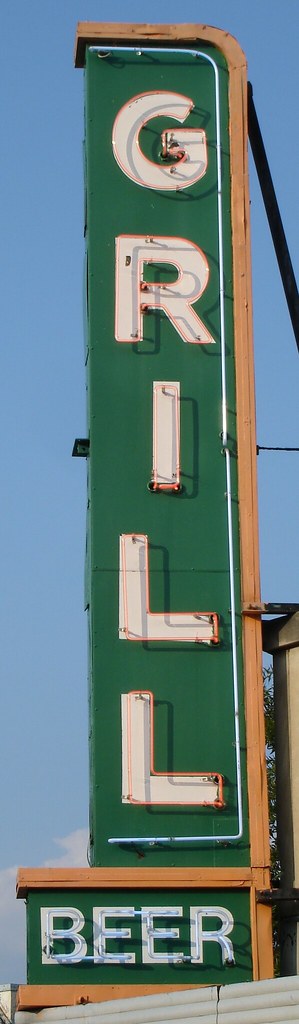This outdoor photograph captures a close-up view of a sign mounted on the side of a building against a backdrop of a clear, blue sky, indicating a sunny day. The sign, designed to be visible to passersby, features a green background with a wooden base. From top to bottom, in light-colored lettering, the word "Grill" is prominently displayed. An outline of neon piping, intended to illuminate the sign at night, frames the lettering, though it is unlit in the daytime setting. Additionally, the word "Beer" runs from left to right at the bottom of the sign, completing the inviting message.